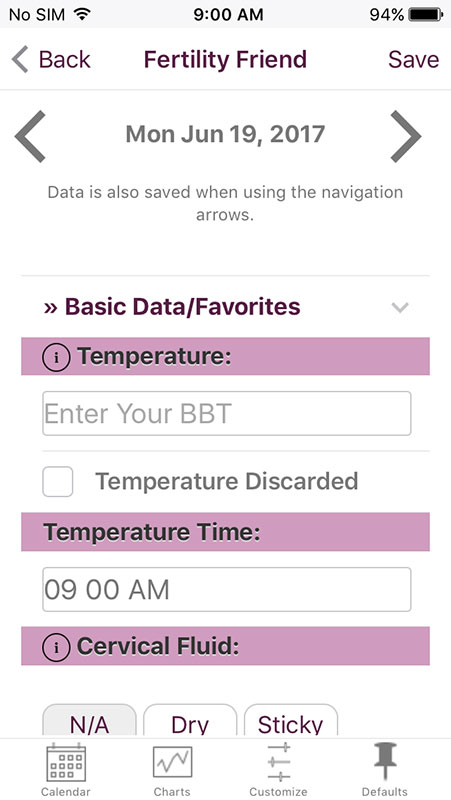A detailed screenshot from a mobile application is depicted. At the top section of the image, the status bar indicates that no SIM card has been inserted while the Wi-Fi signal is fully accessible. The time displayed is exactly 9:00 a.m., and the battery life is at 94%. The application interface has a pristine white background.

Moving down, a navigation bar features a back button on the left, "Fertility Friend" prominently displayed in the center, and a save option on the right. The current date, Monday, June 19, 2017, is displayed with left and right arrows available to toggle between different dates. A note beneath these arrows indicates that data is saved when navigation buttons are utilized.

A purple or pink banner titled 'Basic Data Favorites' partitions the next section, beginning with 'Temperature.' Here, users are prompted to enter their Basal Body Temperature (BBT), with an information icon nearby for further assistance. An option to mark the temperature as 'discarded' is available through a check box, and the temperature entry time is listed as 9:00 a.m.

The succeeding section, highlighted by another pink banner, is dedicated to 'Cervical Fluid' entry. At the bottom of the interface, a fixed navigation bar offers options for 'Calendar,' 'Charts,' and 'Customize' actions, as well as a 'Default' setting marked with a pin icon.